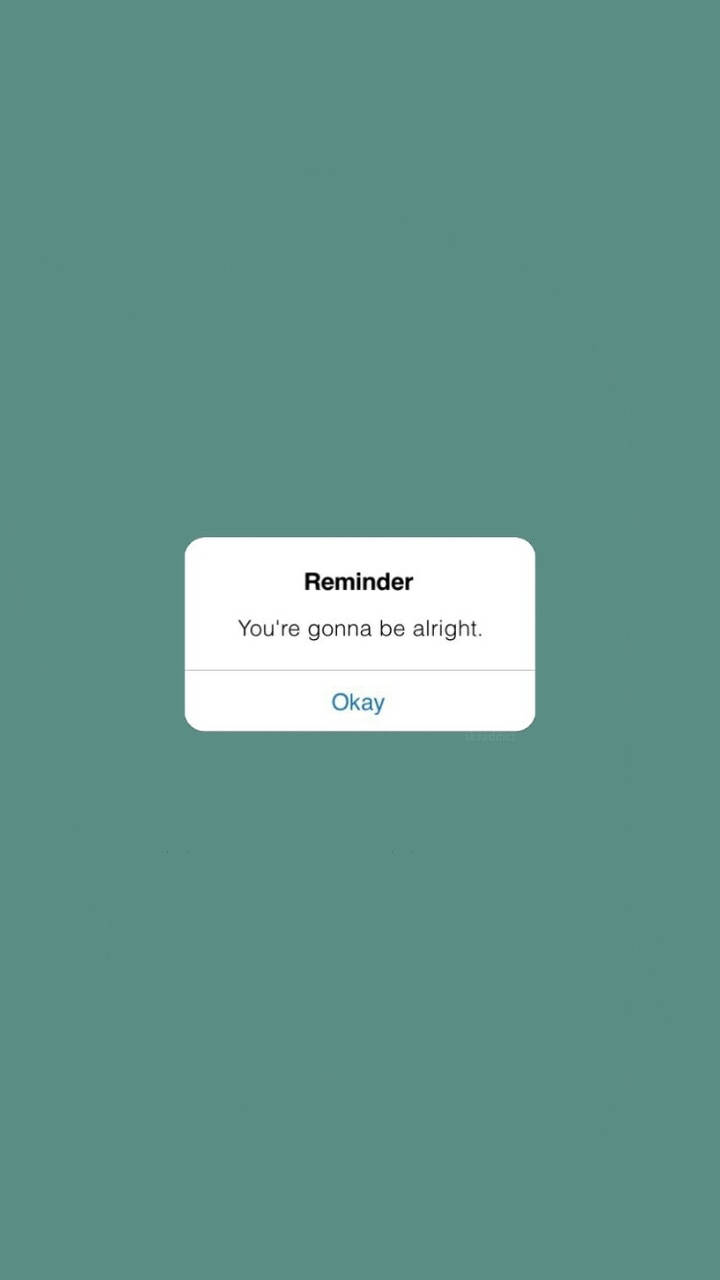The image features a blue gradient background, transitioning from a lighter blue at the bottom to a darker blue at the top. In the center of the image, there is a white rectangular overlay with bold black text that reads, "Reminder: You're going to be alright." Below this reassuring message, a blue button labeled "okay" is prominently displayed.